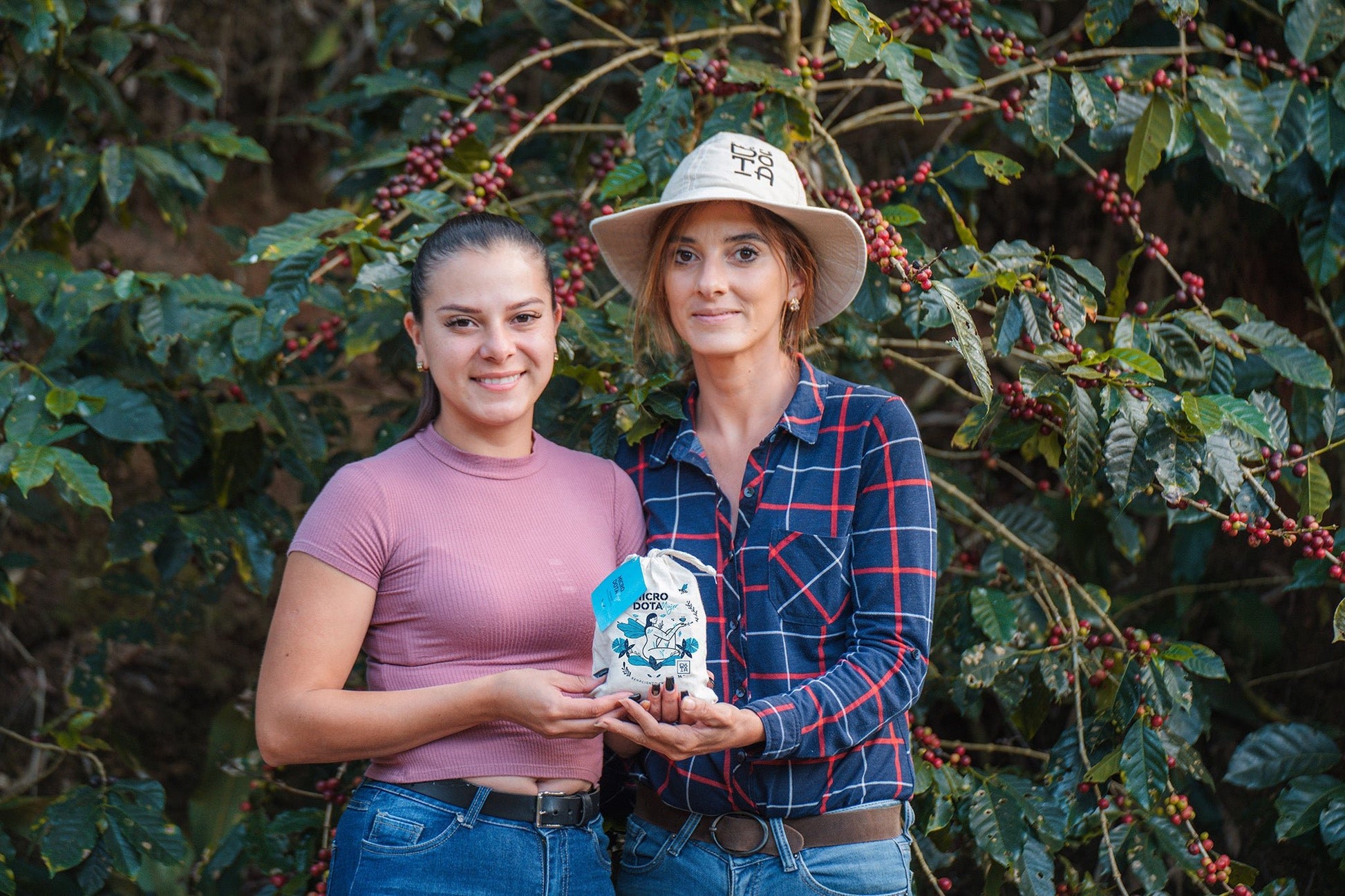This is a realistic, horizontally oriented photograph capturing two Hispanic women from the waist up. Both women are dressed in jeans and brown belts. The woman on the left, who appears to be in her 20s or 30s, has black hair and is wearing a short-sleeved pink top. The woman on the right, also seemingly in her 30s, sports a blue button-up shirt with a red and white plaid design, as well as a white hat. They are gently smiling and holding a bag that has the word "Dota" on it, possibly containing coffee beans or some sort of product associated with the bush or tree behind them, which has green leaves and red berries. The scene appears to be set during the daytime, possibly around sunset, further adding a warm and inviting atmosphere to the photograph.